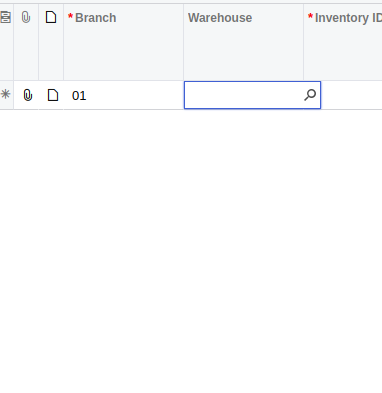A digital form interface is depicted, primarily characterized by a light blue background at the top section. The form is divided into several vertical segments. Starting from the upper left, there is an icon resembling a floppy disk. Adjacent to it, in the next section, is a drawing of a paperclip. Further to the right, another section contains an icon resembling a piece of paper.

Below this, a rectangular section lists the following labels from left to right: "Branch" (preceded by a red asterisk), "Warehouse," and "Inventory ID" (with a red asterisk next to the letter "I"). 

On the bottom row of the form, an asterisk is positioned on the far left. To the immediate right, there is a white-backgrounded area featuring another paperclip icon, a piece of paper icon, and the numeral "01." Further to the right in this row, there is a bright blue-bordered search bar, containing an icon of a magnifying glass within it.